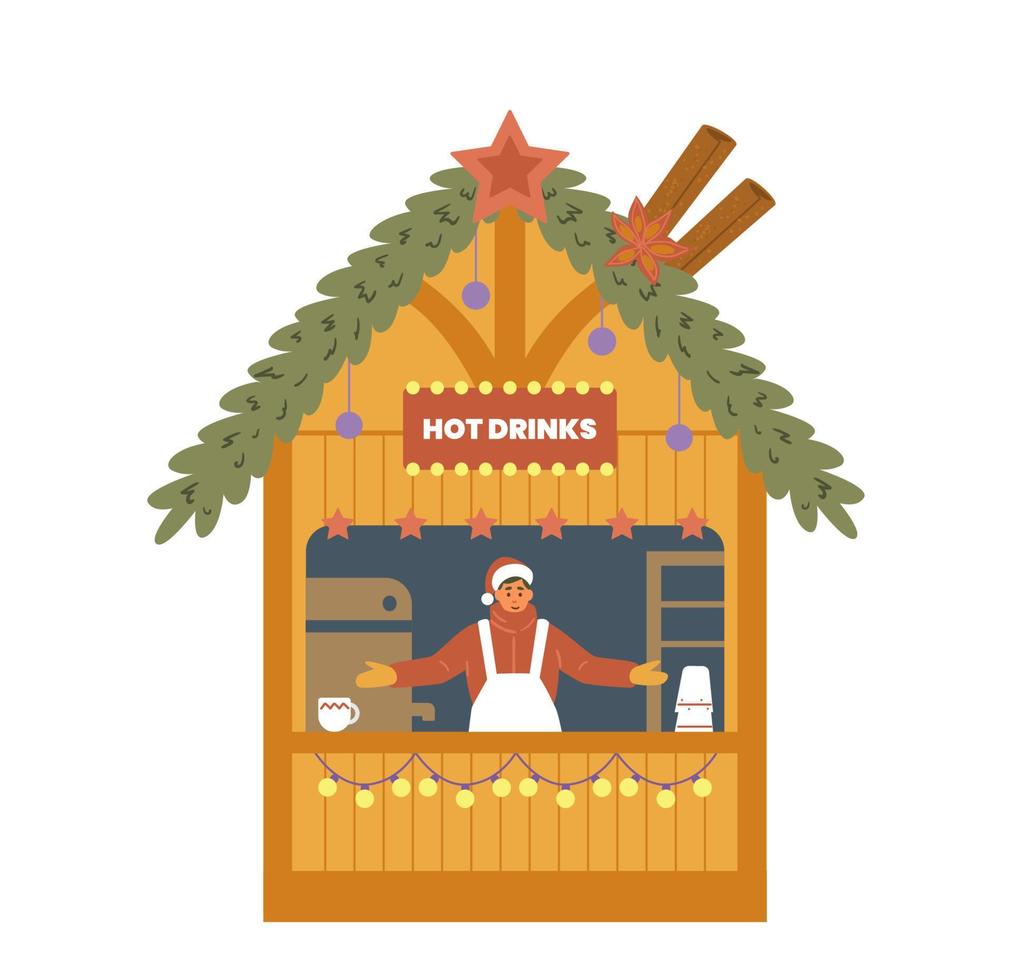This digital artwork depicts a cozy, simplistic drink stand styled as a wooden shack with vertical slats and a leafy roof adorned for the Christmas season. Atop the roof, there are giant sticks of cinnamon and a star, which is red with a smaller red star inside. An orange and yellow flower also sits beside the star. Below, a burnt orange sign bordered by round yellow lights declares "Hot Drinks" in white text. The front of the counter is decorated with teardrop-shaped lights and hanging red stars.

The open serving window frames a male vendor dressed in a festive red sweater with a turtleneck, a white apron, yellow gloves, and a Santa hat. The countertop features a white cup on the left and what appears to be a coffee machine or stack of cups on the right. Behind the vendor, a fridge and shelves are faintly visible, adding to the ambiance of this charming, holiday-themed drink stand.